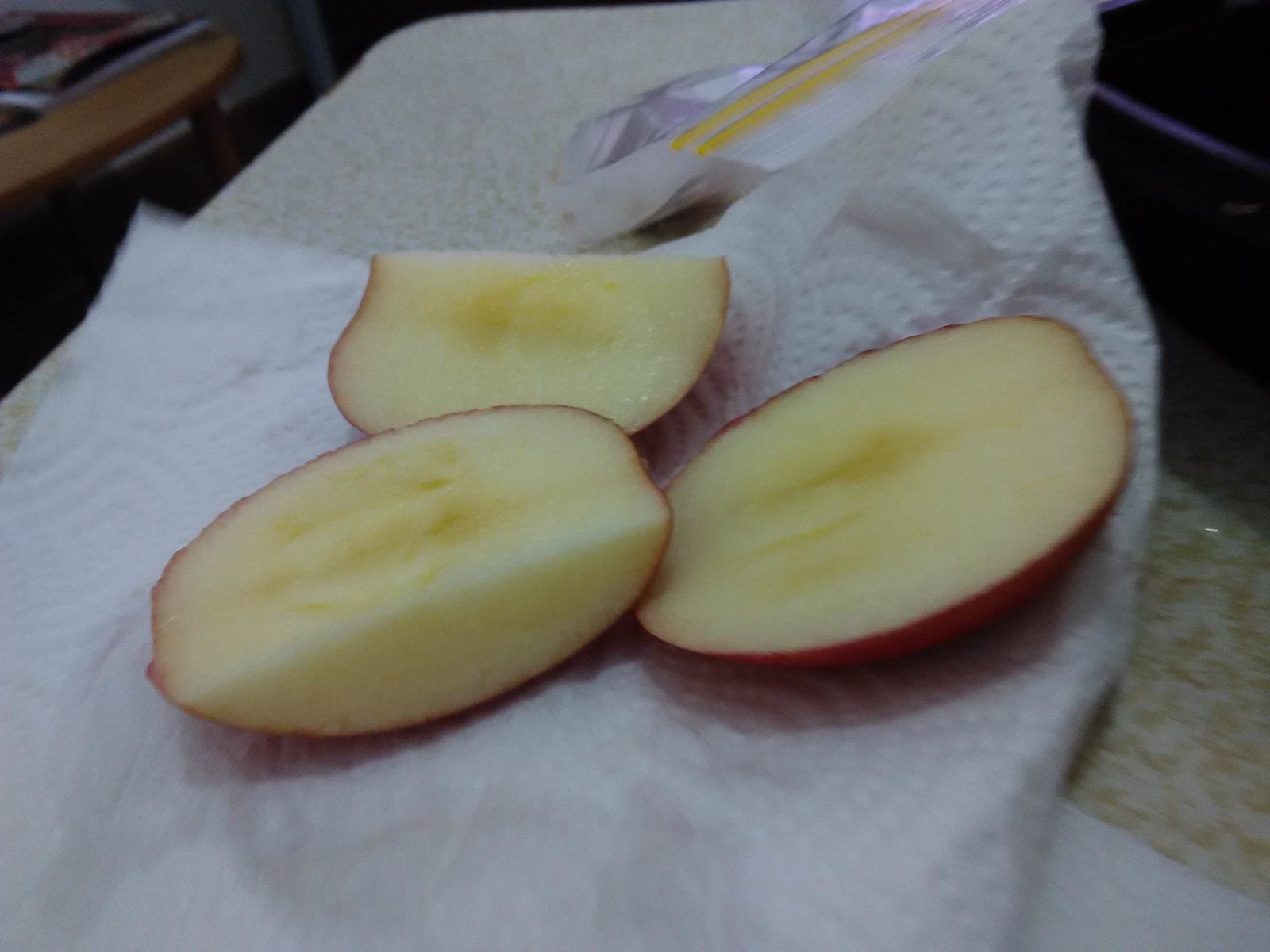In the image, there's a white paper towel laying flat in the middle with what appears to be three pieces of apple on it. The apple slices vary in shape; one is a rounded side slice, another looks like a fourth of an apple, and the third has a half-circle shape. These slices have a reddish peel and beautifully white flesh, with a hint of yellow near the core area. To the right of the paper towel, part of a marble counter is visible, while to the left, a corner of a brown wooden table can be seen. The background has a floral pattern with yellowish-brown hues. A small, white plastic object with two yellow lines is also present on the counter next to the paper towel. The image appears slightly out of focus, suggesting slight movement when it was captured.